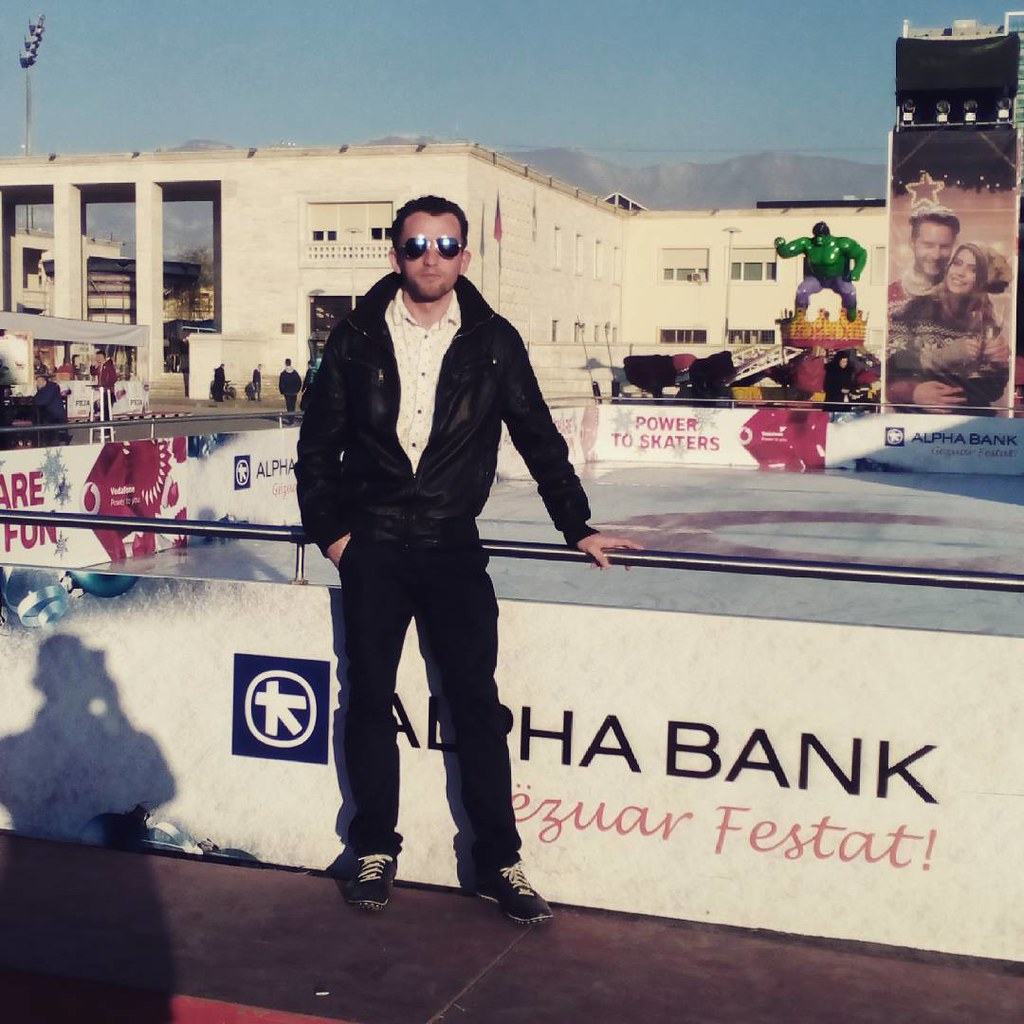This image features a man with short black hair and a goatee, standing on the outside of an outdoor ice skating rink on a sunny day. He is wearing dark-tinted aviator sunglasses, a black jacket, black pants, and black athletic shoes, along with a white button-up collared shirt. He has his right hand resting on a waist-high railing that surrounds the skating rink.

In the lower left of the image, the shadow of the person taking the picture is visible. The background showcases a large white building with open spaces in the middle, as well as an advertisement featuring a woman. To the right of the man and prominently visible in the background is a statue of the Incredible Hulk. Further in the distance, gray, blurry mountains rise under a light blue sky.

Additionally, there are people gathered on the left side of the image, possibly around a table stand, adding to the atmosphere of what appears to be an outdoor fair.